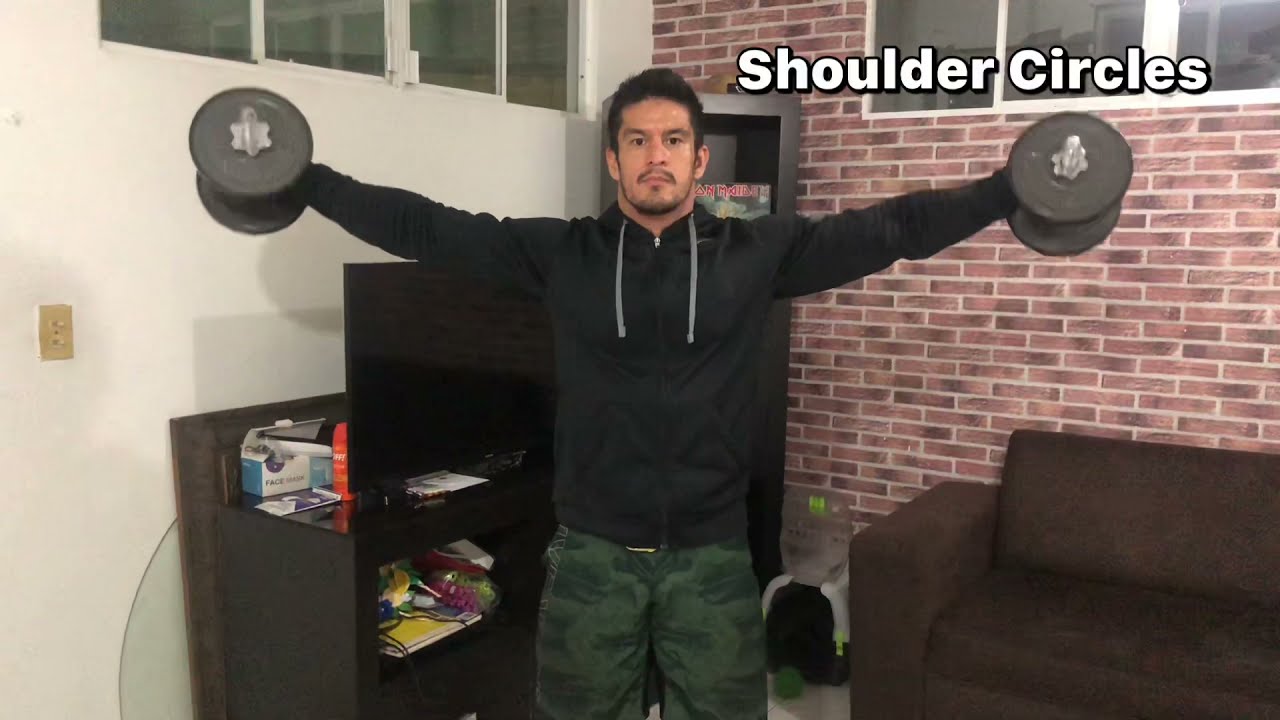A man with dark hair, dark eyes, a mustache, and a beard stands in the middle of the image, wearing a black sweatshirt with gray strings and camouflage pants. He holds a black dumbbell in each hand, extending his arms out to his sides at shoulder level. The room features a brick wall on the right side and a white painted wall on the left, each wall adorned with windows. To his right is a brown couch, and to his left is a television on a stand with various objects around it. Above the man, a caption reads "shoulder circles" in white font with black shadowing.